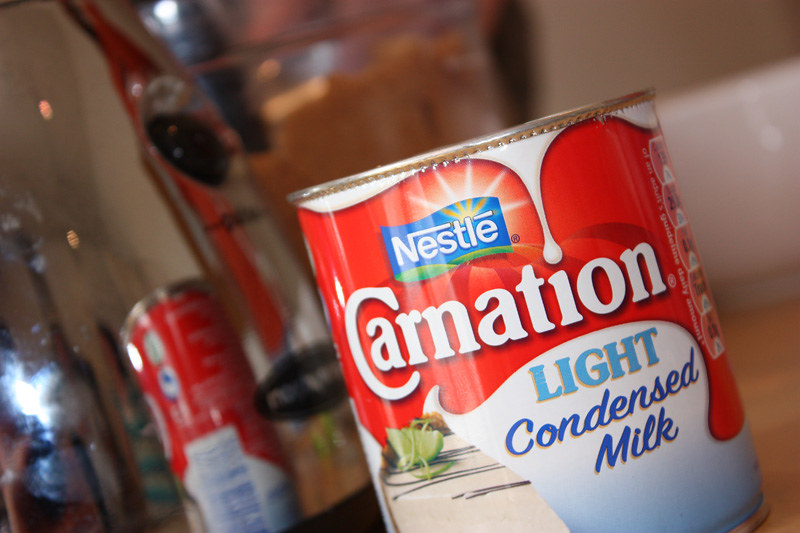This image, taken in a home setting, depicts a can of Nestle Carnation Light Condensed Milk prominently positioned near the center but slightly tilted towards the bottom right corner. The can is angled around 45 degrees. The label features a gradient background transitioning from white to light blue at the bottom, with the iconic Nestlé logo at the top, accompanied by a sun with radiant beams. Below, the word "Carnation" is written in white text against a red backdrop, and "Light Condensed Milk" appears just below it, with "light" in light blue and "condensed milk" in dark blue. A graphic design of milk drips down the sides of the can, adding to its appeal. To the left side of the can, the label appears to tear away, possibly revealing a boat logo. The can is situated in front of a reflective surface, likely a large appliance with a see-through glass top, making the can's reflection visible behind it. Adjacent to the first can, another identical can is partially visible. Both items rest upon a light brown wooden surface.